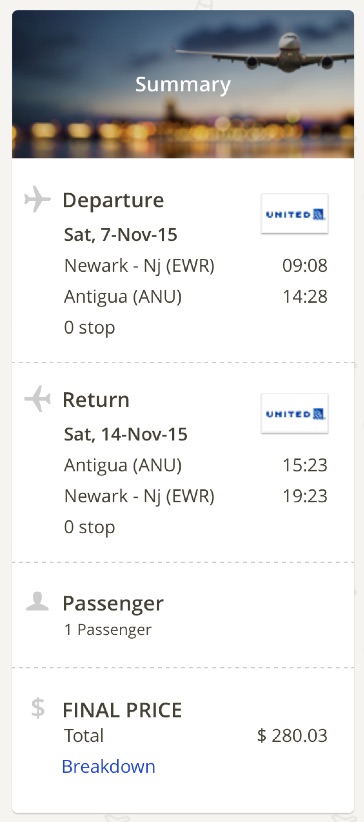The image depicts a detailed summary page on a flight booking website. At the top center, the word "Summary" is prominently displayed in white text. In the background, a white airplane is flying towards the viewer from the top right, against a backdrop that includes a plethora of blurry orange lights. The sky is mostly clear with some dark clouds visible in the upper right corner.

Below this header, the summary is organized into four distinct sections:

1. **Departure Section:** 
   - Date: "Saturday, November 15th"
   - Airline: "United" in a small box
   - From: "New York, NJ, EWR"
   - Departure Time: "09:08"
   - To: "Antigua, ANU"
   - Arrival Time: "14:28"
   - Stops: "Zero stop"

2. **Return Section:**
   - Date: "Saturday, November 15th"
   - Airline: "United" in a small box

3. **Passenger Information:**
   - Specified as "One Passenger"

4. **Final Price:**
   - Total: "$280.03"
   - Labelled with "Breakdown"

This summary provides an overview of the planned flight itinerary, including dates, times, the airline, departure and arrival locations, number of stops, and the total cost.